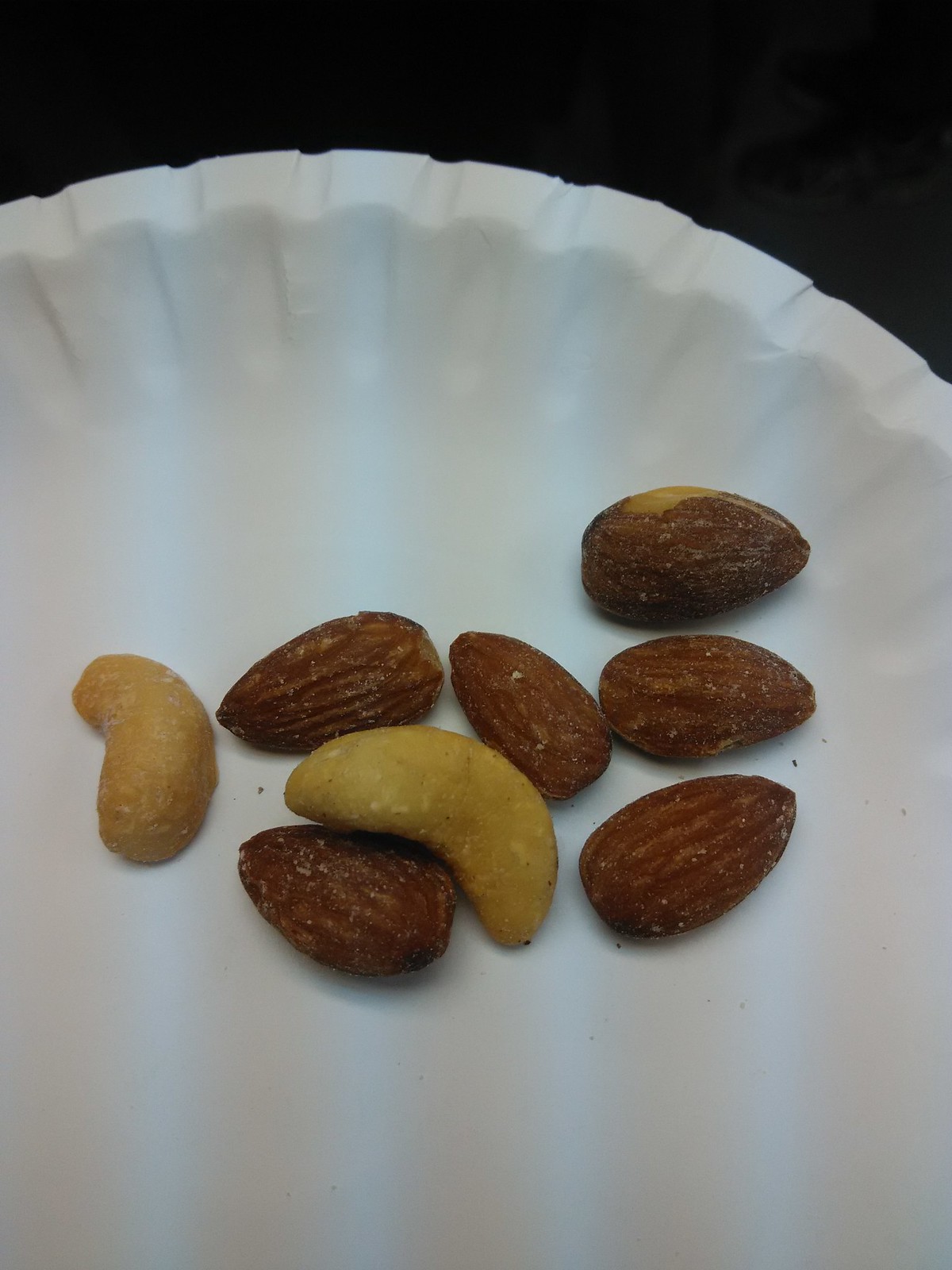This image depicts a close-up of a white paper plate with a small, rigid edge, occupying about 80% of the frame. The plate is set against a black background, which is only about 20% visible. On the plate, there is an assortment of nuts, specifically two yellow cashews and six salted brown almonds. The cashews are positioned with one on the left side and one in the middle of the plate. The almonds are arranged such that three of them are vertically aligned to the right of the middle cashew, with their narrower ends pointing right. The remaining three almonds nestle around the middle cashew, complementing its shape. The nuts appear to be seasoned with a white, salt-like substance. Only the edge of the plate on the upper one-fourth of the image shows a hint of purple.